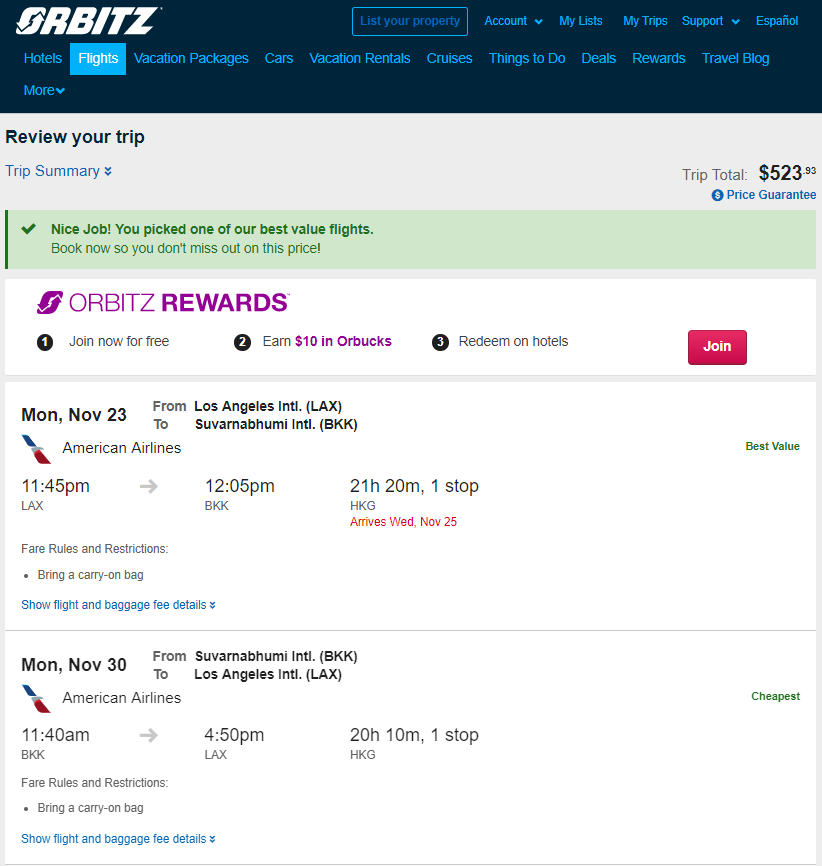Screenshot of a Travel Booking Website with Orbits Branding

This is a detailed screenshot of the Orbits travel booking website. The overall background of the page is a dark blue, contrasted by lighter blue text. At the very top, the Orbits logo is prominently displayed. Below the logo, navigation options are listed in a horizontal line with dark blue text on a light blue background. The options include "Flights", "Hotels", "Vacation Packages", "Cars", "Vacation Rentals", "Cruises", "Things to Do", "Deals", "Rewards", and "Travel Blog".

A light blue rectangle with white text highlights the "Flights" section, indicating it is the current focus of the page. Under this navigation bar, in white text on a light blue background, is a summary of the trip cost, stating "Trip Total: $523.83". 

Below the trip total, there's an icon of a blue circle with a white dollar sign inside, accompanied by blue text that reads "Price Guarantee". Nearby, a red rectangular button with white text prompts users to "Join". Adjacent to this, purple text in all caps announces "ORBITZ REWARDS".

Further down, there is a black circle with a white number "1" inside it, with the black text next to it stating "Join Now for Free". The call-out sections in green text highlight offers: one labeled "Best Value" and another labeled "Cheapest". 

Finally, there's blue text that resembles a hyperlink, which reads "Show Flight and Baggage Fee Details", inviting users to click for more information.